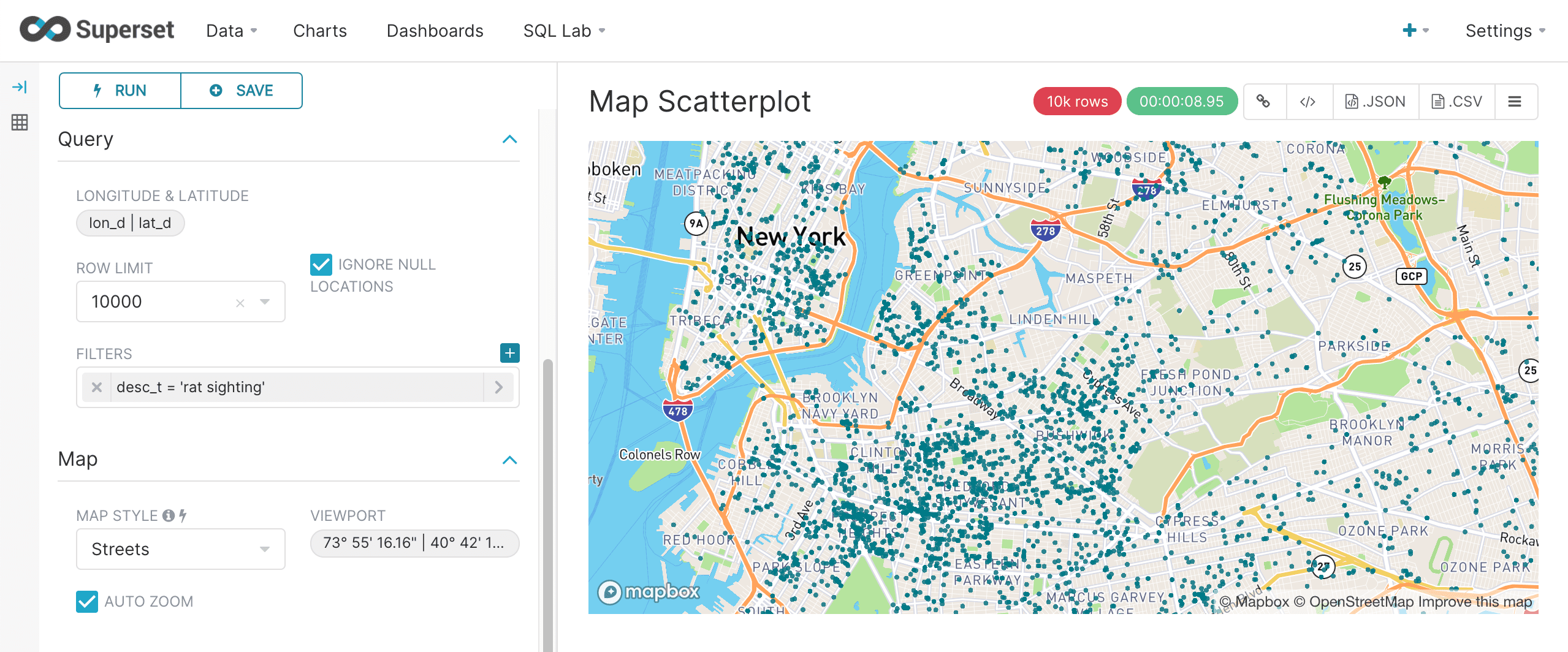This is a screenshot capturing a comprehensive website layout. 

Across the top, the website features a white border followed by a thin gray line. On the left side, there's a half-inch gray border, transitioning to a white section that spans about one-third of the page width. Further down, the area consists of one inch of white space, followed by two inches of light gray, and then another two inches of dark gray. Adjacent to these sections, a detailed map is displayed.

In the top left corner of the interface, there's an infinity symbol with a blue center and black edges. The bolded text next to it reads "Superset," followed by regular font labels: "Data," "Charts," "Dashboards," and "SQL Lab." On the right side, the word "Settings" is positioned, while to its immediate left, there's a blue plus sign.

To the left within the white border, two white tabs with blue borders are visible. The left tab reads "Run" and the adjacent one reads "Save." Below these tabs, the word "Query" appears in black. Further down, fields for entering limits, longitude, and latitude, along with filters, are present. Following this, the heading "Map" is displayed in black, succeeded by "Map Style: Streets."

On the right side, information labeled "VFW Port" is present, describing details about it. In the bottom left corner, a blue square with a white checkmark labeled "Auto Zoom" can be found. Above the map, the heading "Map Scatterplot" appears in black text. A red tab labeled "10K rows" and a green tab displaying "00:08.95" are located towards the middle of the screen.

Further down, five white tabs are present. The first tab features a chain link symbol. The second tab has a greater-than sign pointing both left and right, with a slash in the center. Subsequent tabs are labeled "JSON," "CSV," and one featuring three horizontal lines.

The map below these elements is of New York. It shows water bodies along the left and top boundaries, with grayish and some green landmasses. Blue pins are scattered densely across the map, along with three or four orange lines denoting roads.